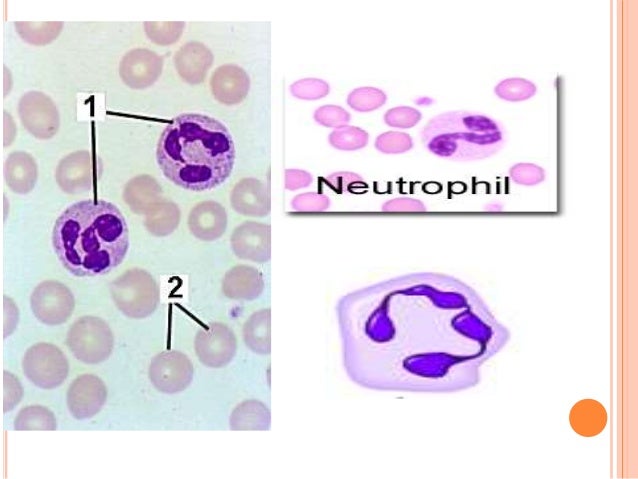This detailed image depicts cells as viewed under a microscope against a white background. On the left, there is a blue rectangular section featuring cell structures. Two dark purple circles, each with an even darker spot, are labeled with a white square containing the number '1'. Black lines extend from this number to the circles. Beneath this, the number '2' connects to two smaller, light purple circles. 

On the right side, the word "neutrophil" appears in light purple text accompanied by dark purple designs and multiple circular elements. Below this, an off-circle shape with intricate dark purple or blue patterns is present. Finally, in the bottom right corner, there is a prominent orange circle. This poster thoroughly categorizes the cells, highlighting the neutrophils and other cellular components through a series of distinctive visual aids and labels.